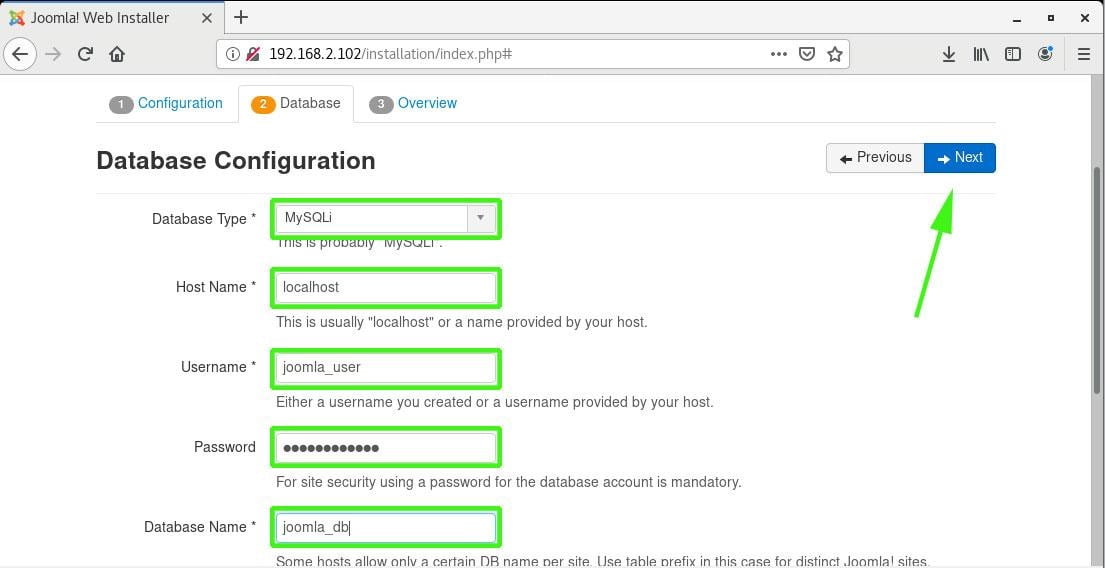### Detailed Caption:

This image is a screenshot of a computer screen displaying a web browser tab labeled "Joomla! Web Installer." The tab description is followed by a close button (an 'X') and a plus button for opening a new tab. On the browser's right side, there are controls: a minimize button, a button for adjusting window size, and a close button. Additionally, there are navigation buttons: a back button, a grayed-out forward button indicating there's no page to navigate forward to, followed by a refresh button and a home button.

In the browser's address bar, a red lock icon with a line through it indicates an unsecured connection, and the URL displayed is `http://192.168.2.102/installation/index.php`. Next to the URL are an unknown pound sign (#), three horizontal dots, a check mark, and a star icon.

The Joomla! Web Installer interface within the browser contains three tabs for the installation process: "Configuration" (marked with a gray '1'), "Database" (marked with '2' and currently selected), and "Overview" (marked with '3'). Beneath these tabs are navigation buttons: "Previous" and "Next."

The "Database" tab includes several fields for database setup:
1. **Database Type**: Set to `mysqli`
2. **Host Name**: Set to `localhost`
3. **Password**: Displayed as a series of black dots for security
4. **Database Name**: Set to `joomla_db`

This detailed setup guide indicates the user is in the midst of configuring a Joomla! installation, specifically working on the database connection settings.